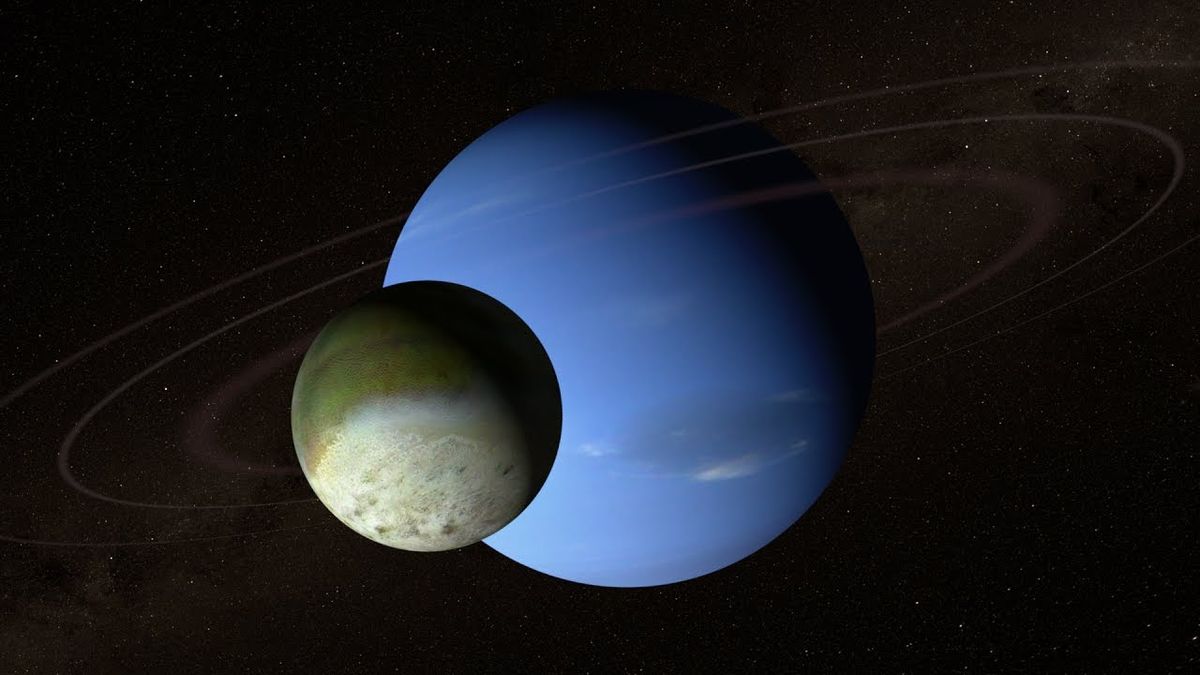The image is a computer-generated graphic showcasing a cosmic scene. At its center is a large blue planet adorned with three faint, light gray rings encircling it. Approximately three-quarters of this planet is visible, with the remaining portion shrouded in shadow. Notably, in the lower right-hand corner of the blue planet, there's an oval-shaped spot of brown or gray hue. 

Adjacent to this planetary giant, on its left, is a smaller celestial body—likely a moon. This moon, approximately one-third the size of the blue planet, features a mix of yellow, green, and white coloration and is partially illuminated, presumably by a nearby star. Both celestial objects are set against a dark, black expanse peppered with tiny white speckles, representing distant stars, giving the entire scene a distinctly outer space ambiance.